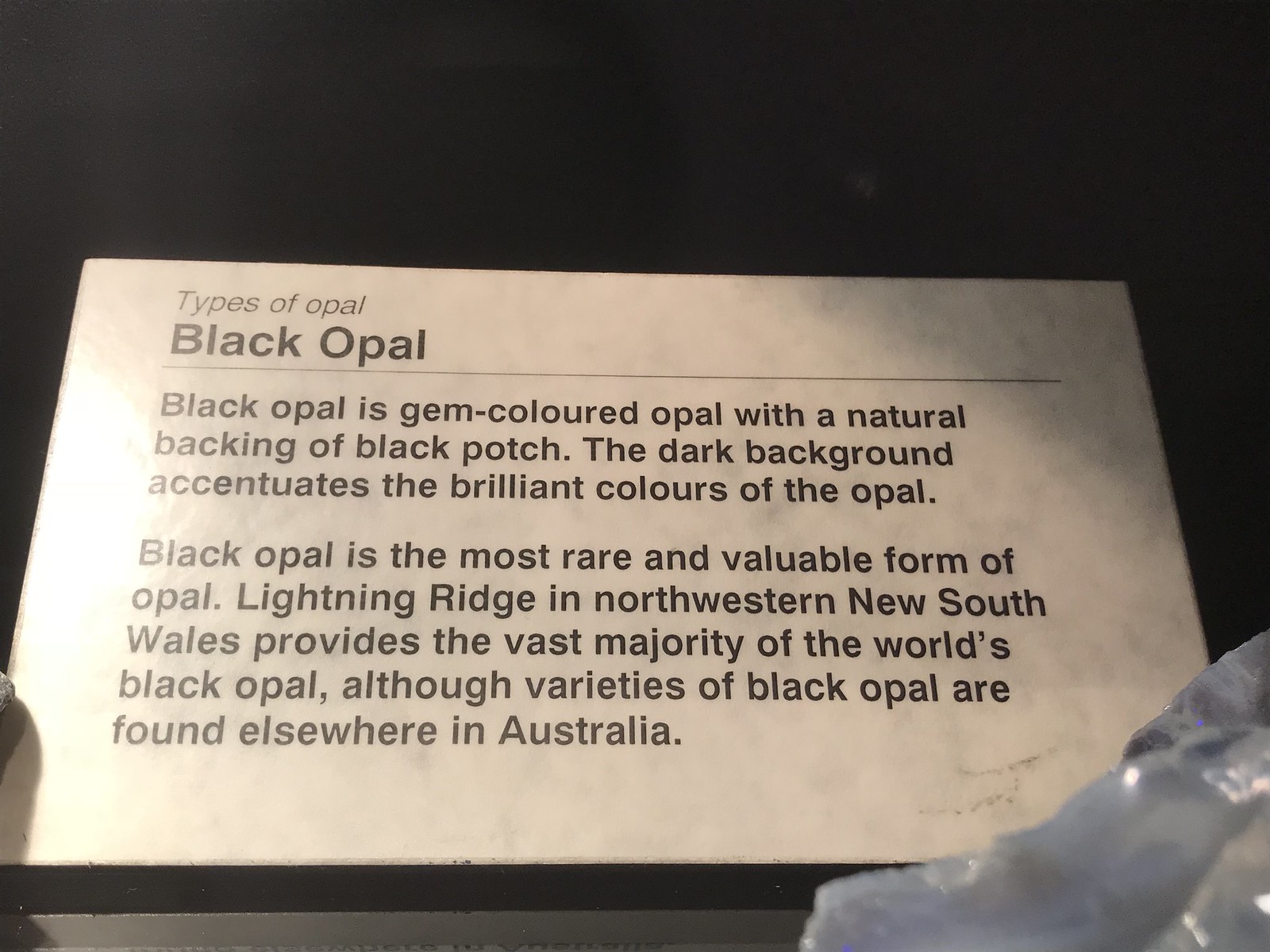The image captures an indoor display, likely from a museum or natural history exhibit, featuring an information plaque about black opal. The plaque is beige with mottling, suggesting it could be composed of stone or simply weathered from long-term exhibition. It prominently reads "Types of Opal" followed by a section on "Black Opal," detailing that black opal is a gem-colored opal with a natural backing of black potch. Noted for being the rarest and most valuable form of opal, it primarily comes from Lightning Ridge in Northwestern New South Wales, though other varieties are found throughout Australia. The plaque is positioned slightly elevated in the upper left-hand corner of the image, with a bright light source enhancing its presence against the predominantly dark background. In the lower right corner of the image, there is a crystal-like, translucent rock, possibly a sample of black opal, whose brilliant colors are accentuated by the dark surrounding. The contrasting light and shadow further highlight the details in both the rock and the informational plaque.